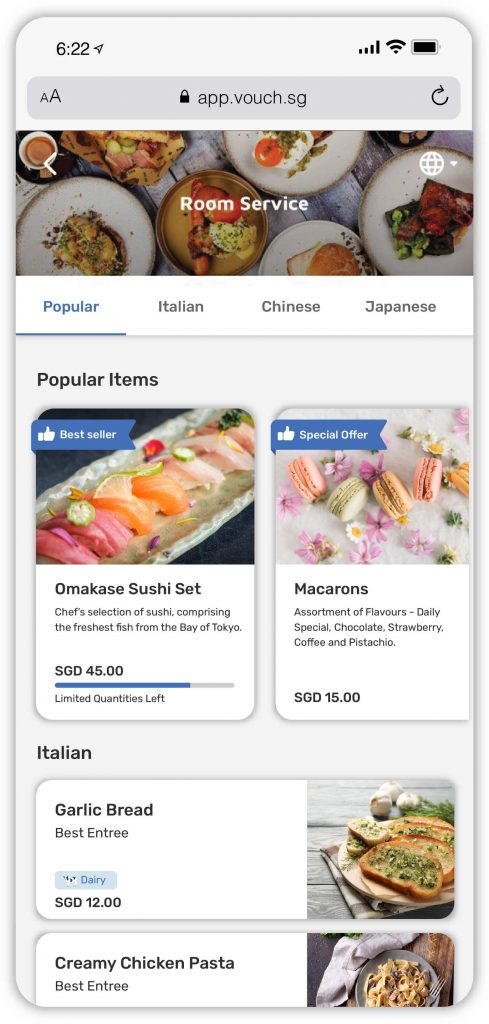The image appears to be a screenshot from a smartphone, displaying a food ordering app labeled "AppVouch.sg" at the top. The status bar indicates the time as 6:22, with icons showing a strong Wi-Fi signal, a fully charged battery, and full service bars. Below the status bar, the app showcases food options under a section titled "Popular Items." 

The main image features several plates of food with the text "Room Service" overlayed in white. One highlighted dish is the "Amakas Sushi Set," which includes pink fish, salmon, and possibly tuna. It's marked as a "Bestseller." 

To the side, there's a special offer for macaroons, described as an "Assortment of flavors," including daily specials like chocolate, strawberry, coffee, and pistachio, accompanied by an image of colorful macaroons. Further down, the menu lists additional items including "Italian Garlic Bread" and "Creamy Chicken Pasta."